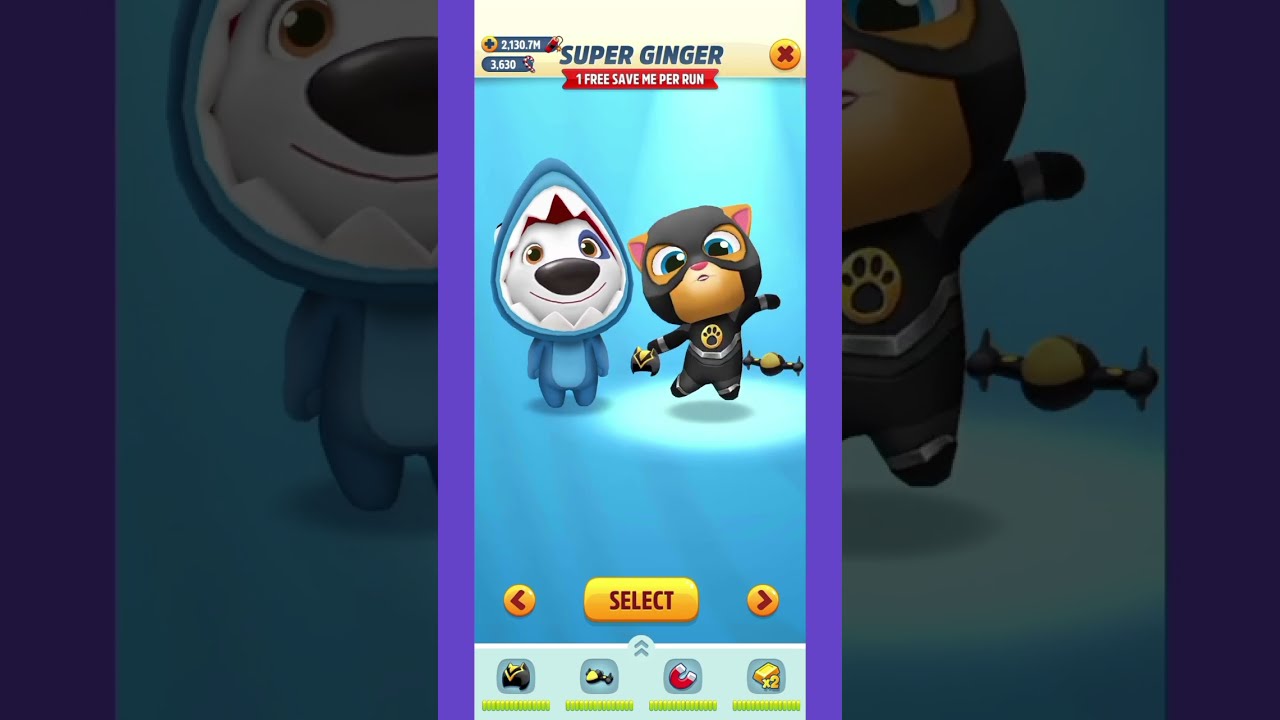In this screenshot of a video game interface resembling "Secret Life of Pets," we see two costumed animal characters. At the top of the screen, a light yellow bar displays a plus sign with "3130.7M" next to it and "3610" beneath. Centered in blue text is "Super Ginger," followed by a red banner with white text stating "one free save me per run." To the right, there's an orange circle with a cross mark in it.

The character on the left is a white dog with a black nose, wearing a shark costume that has its mouth open, revealing the dog’s face. The dog’s costume features a mix of light and dark blue colors. The cat character to the right resembles Batman, with a black and gold costume bearing a yellow paw print emblem on its chest. This cat has its arms outstretched and legs bent off the ground. Beneath them is a large, bright circle on a mostly light blue ground.

At the bottom center is a gold bar labeled "select," flanked by arrows pointing left and right. Below this are four small symbols, including a red magnet and an item resembling cheese. Purple bars are visible on either side of the symbols. Additionally, the left and right sides of the screen show zoomed-in sections of the respective characters: the dog on the left and the cat on the right, with the background featuring light blues and purples. The overall design suggests this is the character selection screen of a vibrant, colorful video game, possibly for mobile devices.